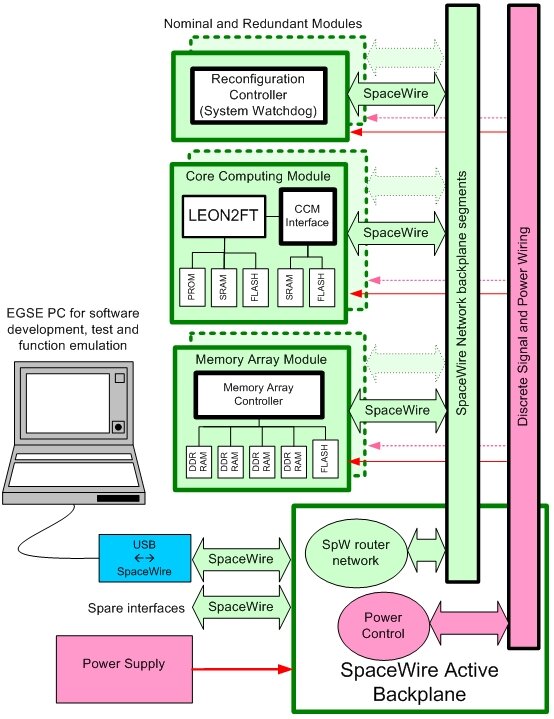The image is a detailed diagram depicting the architecture and connections of a computer-based system, likely related to software development, test, and function emulation. At the top, the diagram is categorized into "Normal" and "Redundant Modules." It features a series of interconnected boxes with space wire connections running vertically down the center. 

1. The top box, labeled "Reconfiguration Controller System Watchdog," oversees system stability.
2. The next layer is the "Core Computing Module (CCM)," which includes a module labeled "LEON2F2" feeding into the "CCM Interface" with two outgoing connections, while LEON2F2 itself has three outgoing connections.
3. Beneath the CCM, there's a "Memory Array Module" managed by a "Memory Array Controller" displayed in a black box, from which five connections extend.

The space wire network and backplane segments are enclosed in a blue box, connecting to discrete signals and power wiring highlighted in pink. Toward the bottom, "Space Wire Active Backplane" and "SPW Router Network, Power Control" manage the overall connectivity and distribution of power. 

A USB space wire from this structure leads to an illustrated gray laptop labeled "EGSE PC for Software Development, Test, and Function Emulation." Finally, there's a "Power Supply" that feeds energy into the entire system. The diagram is color-coded, with light green and hot pink sections denoting different types of wiring and control modules, providing a visual guide through the system’s complex architecture.